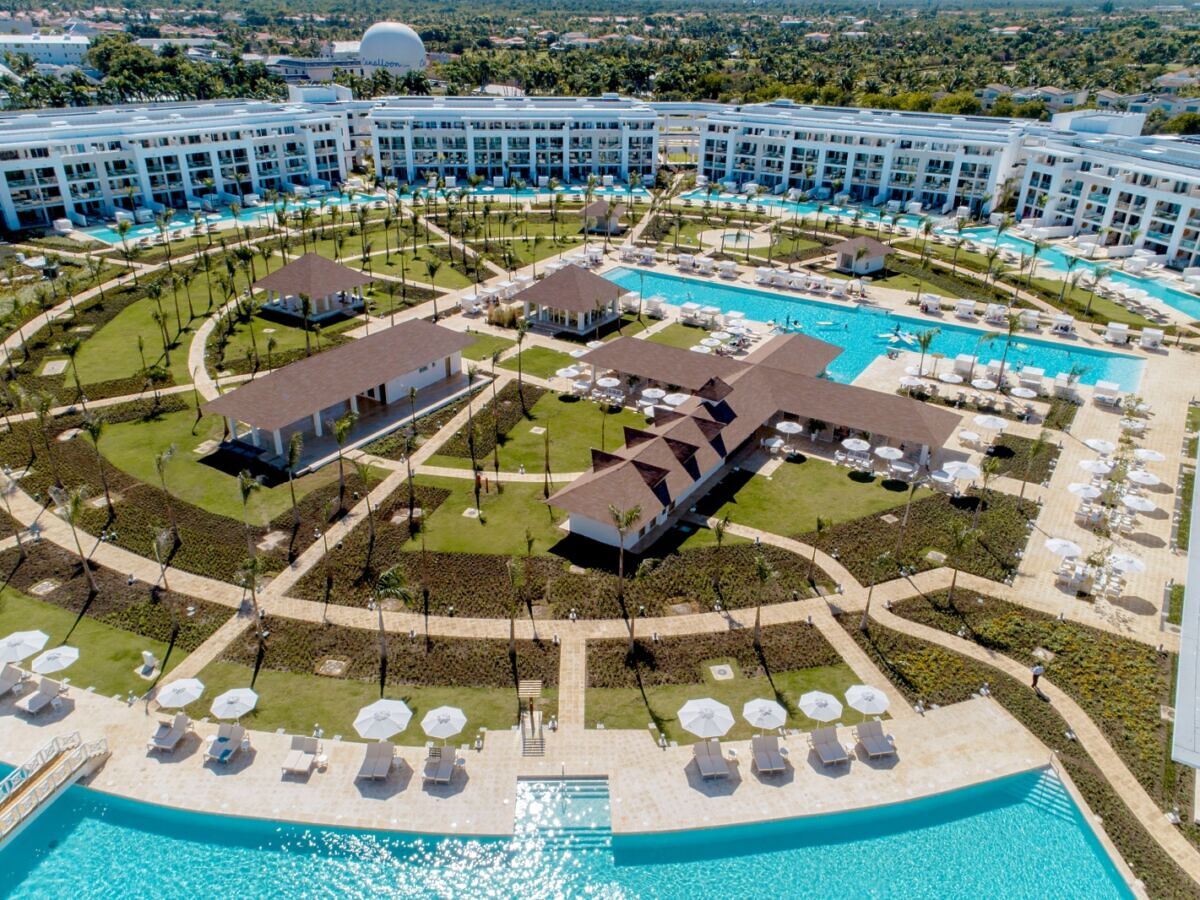The photograph showcases an aerial view of an expansive, circular-shaped resort surrounded by dense green vegetation and various types of trees. The outer perimeter features four large, white buildings with many windows, arranged in a half-semicircle. Inside this semicircle, tan-colored walkways encircle the resort's interior, which includes multiple bright blue swimming pools, one notably in the foreground. Scattered throughout the interior are white pool chairs with matching umbrellas. At the center, there is a distinctive cross-shaped building, flanked to the left by a long, rectangular building, and accompanied by several smaller structures including gazebos and square buildings. The area also features a green and dark brown field with mulch and plants, enhancing the elegant landscaping of the resort.